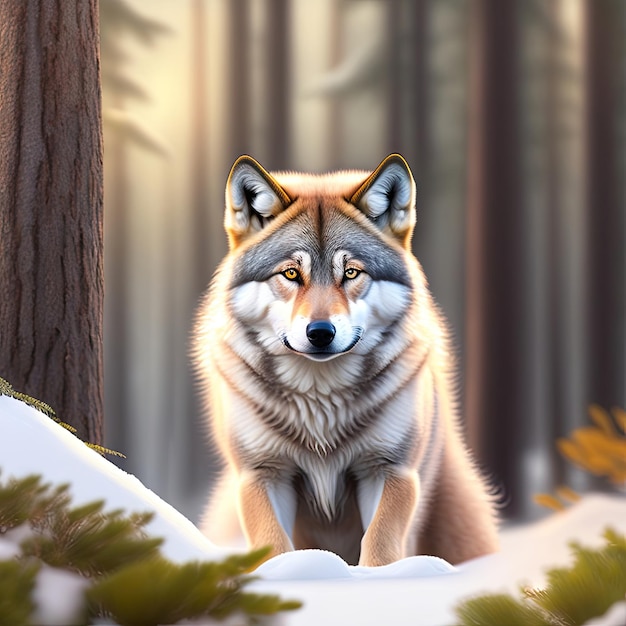The image appears to be AI-generated or artist-rendered rather than a photograph. It features a striking depiction of a wolf, or a similarly wild canine, prominently in the center, staring directly at the viewer with neutral, slightly piercing yellow or hazel eyes. The wolf's fur showcases an intricate mix of white, cream, brown, and dark grey hues, with a symmetrical face, a black nose, and distinctive markings across its snout and head. The ground is covered in pristine white snow, accented by green plants poking through. To the left, a textured tree trunk adds depth, and the background fades into a foggy blur of tall, snow-dusted trees, enhancing the sense of wilderness in the scene.